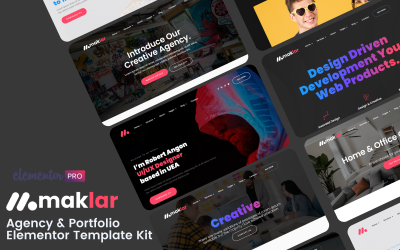The image features a gray background with distinctive elements. In the bottom left corner, "Elementor" is written in elegant purple cursive script. Adjacent to it, there is a magenta-colored box labeled "Pro." Directly beneath these, two white diagonal lines and a circle frame the text. The letters "M-A-K" are prominently displayed in white, while "L-A-R" follows in purple. Below this, the phrase "Agency and Portfolio Elementor Template Kit" is rendered in gray letters.

The central portion of the image showcases a series of diagonally aligned, tightly packed boxes with various images and text. Among them, one box features the phrase "Introduce Our Creative Agency." Another box presents an image of a man wearing a hoodie, accompanied by the text "I'm Robert Angon, UX Designer based in USA." Below that, another box simply states "Creative."